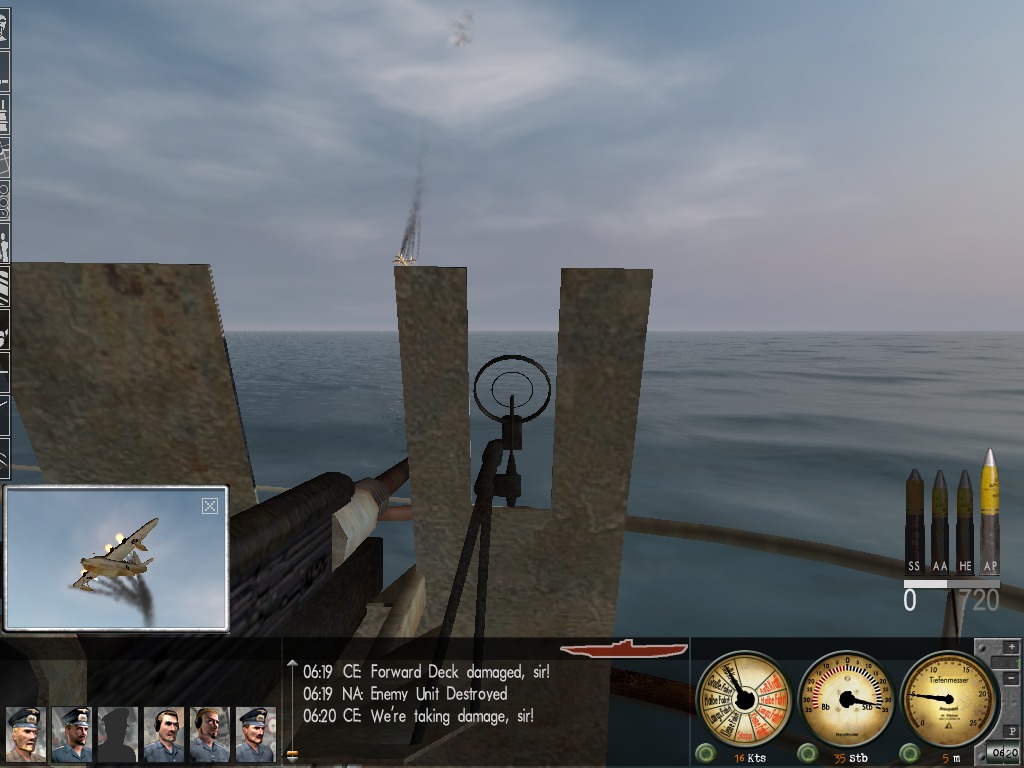This is a detailed screenshot from a computer game set during World War II. The image features the perspective from the deck of a boat, looking through the sight of a machine gun. In the distance, a warplane, which appears to have just been shot down, trails black smoke as it plummets towards the ocean. The sky is a grayish-blue, filled with thin clouds, contributing to the dreary atmosphere. 

To the left of the main viewfinder, there is a small in-game thumbnail showing an undershot of the downed white-finished airplane amidst flames. On the right-hand side of the screen, there are illustrations of missiles or bullets, emphasizing the ongoing battle. Below these illustrations, three gauges whose exact purposes are unclear provide additional game data.

The bottom part of the screen features several key elements. The lower-left corner displays six squares, with five containing pictures of soldiers and one merely showing a black silhouette, indicating player avatars. In the middle of the bottom portion, critical game status texts are visible: "619 CE forward deck damage, sir,” "619 NA enemy unit destroyed,” and "620 CE we're taking damage, sir.” Above this text on the right side is an outline of a red boat, possibly indicating the player's vessel.

In summary, the screenshot captures the tense moment of naval warfare in the game, with vivid details highlighting the aircraft's downing, combat status updates, and different interface elements providing essential information for the player.